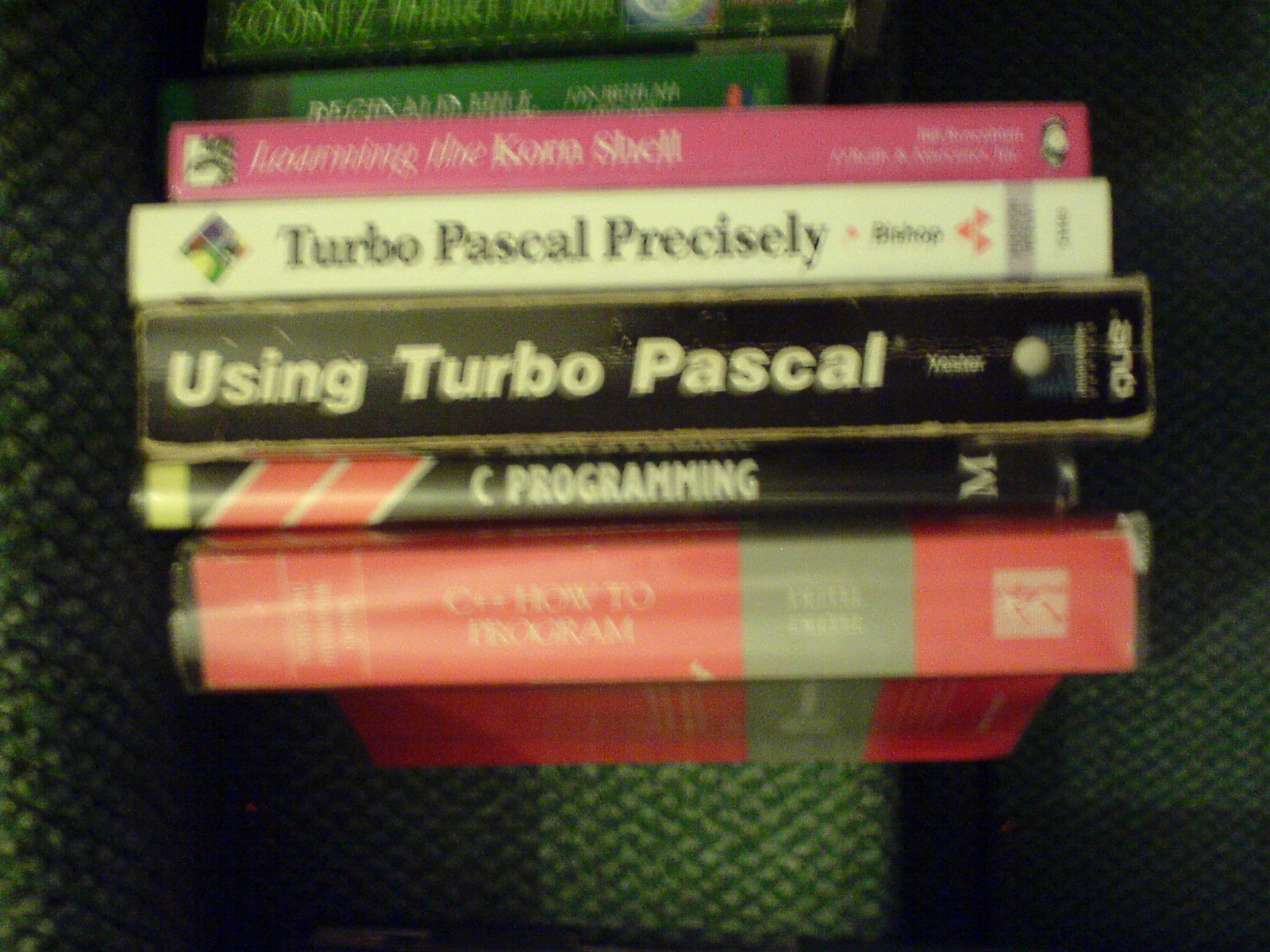This image is a slightly blurred photograph of a stack of books, viewed from above, with their spines facing outward. The spines show an array of colors including red, black, white, pink, and dark green, each indicating different sizes and thicknesses of the books. Despite the blur, some titles are discernible such as "Using Turbo Pascal," "C Programming," and "Turbo Pascal Precisely," suggesting the books are related to computer programming. The books seem to be resting on a piece of fabric or carpet which is also slightly out of focus, showing a mix of darker and lighter stripes and patches in green, white, and other muted tones.